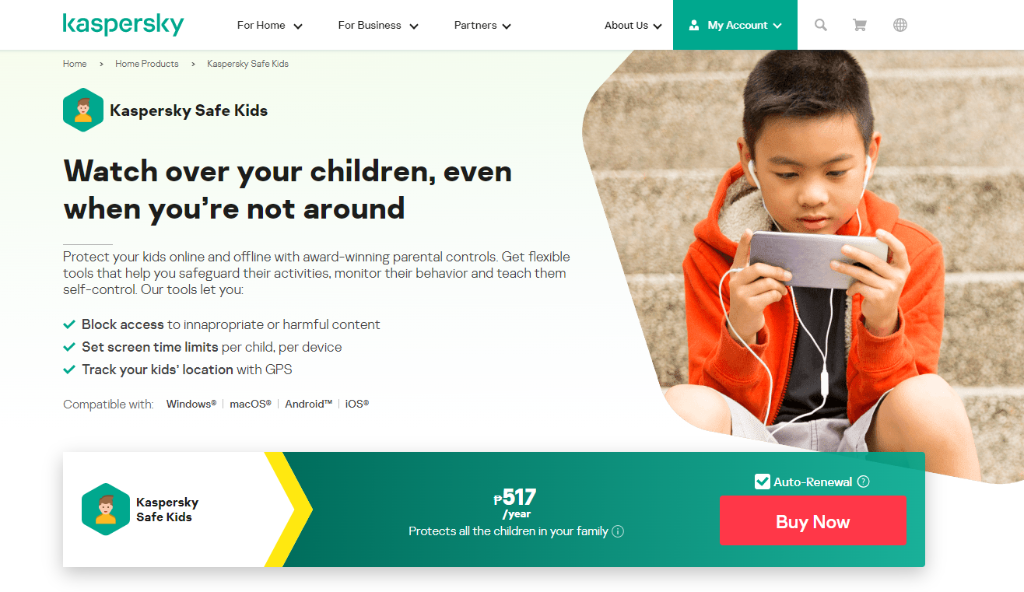This is a detailed screenshot from the Kaspersky website, prominently featuring their "Safe Kids" product. At the top left, the header displays "Kaspersky" in green text. To the right, there are clickable sections labeled Home, For Business, Partners, About Us, My Account, along with icons for search, a shopping cart, and a globe symbol.

Below the header, there are breadcrumb links: Home, Home Products, and Safe Kids, indicating the page's location within the site. The Safe Kids logo is displayed nearby, depicting a small human figure within a green octagon.

Adjacent to the logo, the text "Kaspersky Safe Kids" is written again. Underneath, a bold statement in black text reads, "Watch over your children even when you're not around." This is followed by a smaller paragraph describing the product's features: "Protect your kids online and offline with award-winning parental controls. Get flexible tools to help you safeguard their activities, monitor their behavior, and teach them self-control. Our tools let you block access, set screen time limits, track your kid's location."

An image illustrates a child using a phone with headphones connected to the device and in his ears, visually emphasizing the product's focus on safeguarding children’s digital activities.

At the bottom of the screenshot, the Kaspersky logo appears again alongside the product's price, and buttons to enable auto-renewal and purchase the product now.